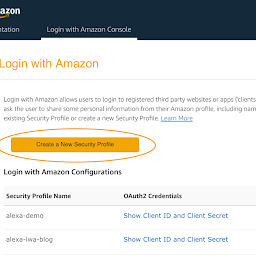The image depicts a partial screenshot of the Amazon Login Console interface. At the very top, a black border is visible. In the upper left corner, the truncated text "A-Z-O-N" can be seen, hinting at the partial presence of the Amazon logo along with a fragment of the iconic yellow smiley face.

To the right, the text "Log in with Amazon Console" is prominently displayed. Below this, a white background section contains further text in yellow, which reads, "Log in with Amazon." Accompanying this is a detailed description that states, "Log in with Amazon allows users to log in to registered third-party websites or apps." It further explains, in parentheses, "Clients ask the user to share some personal information from their Amazon profile including name, existing security profile, or create a new security profile."

There is also a blue text link labeled "Learn more." Below this informational text, an orange button with the label "Create a new security profile" is highlighted and encircled by a yellow oval.

Further down the page, the text "Log in with Amazon Configurations" introduces two main sections: "Security profile name" and "Queue authorization to credentials." Within these sections, two profile names are listed: "Alexa Demo" and "Alexa IWA Blog."

To the right of each profile name, there are blue links labeled "Show client ID and client secret," indicating these options provide further credential details.